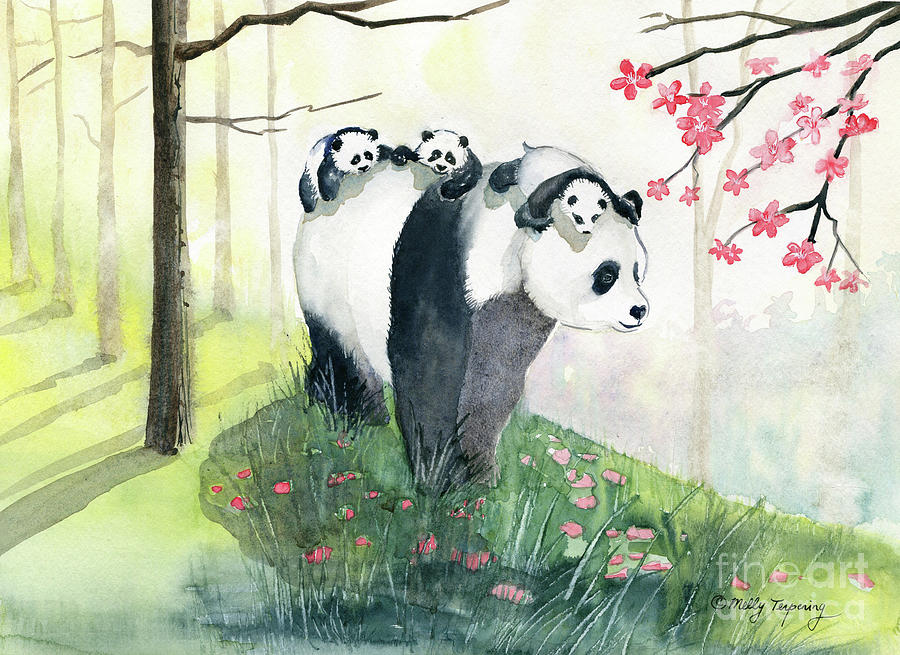The watercolor painting, presented in a horizontal rectangular format, meticulously depicts a mama panda bear with three baby pandas clinging to her. Standing next to a white wall, the mama panda has a white face with black eye patches, a black heart-shaped nose, black ears, and both black front and rear legs. Her body has white fur across her neck and upper back. Of the three baby pandas, one is perched atop her head, another is positioned in the middle of her back, and the third clings precariously to her rear. Each baby panda mirrors their mother with black eye patches, white bodies, and black limbs.

The scene is vibrant and full of detail: the panda family stands on a patch of dark green grass speckled with red and pink flowers. To the right, a tree limb adorned with pink cherry blossoms stretches into the scene, while on the left, several bare trees create a striking contrast. Additionally, scattered flower petals are visible on the ground. High above, a central light source illuminates the painting, enhancing its rich colors. 

In the bottom right corner, the artist's signature, Millie Taiping, is present, along with a watermark reading Fine Art America. The artwork's overall style suggests it is a refined example of Chinese watercolor painting.